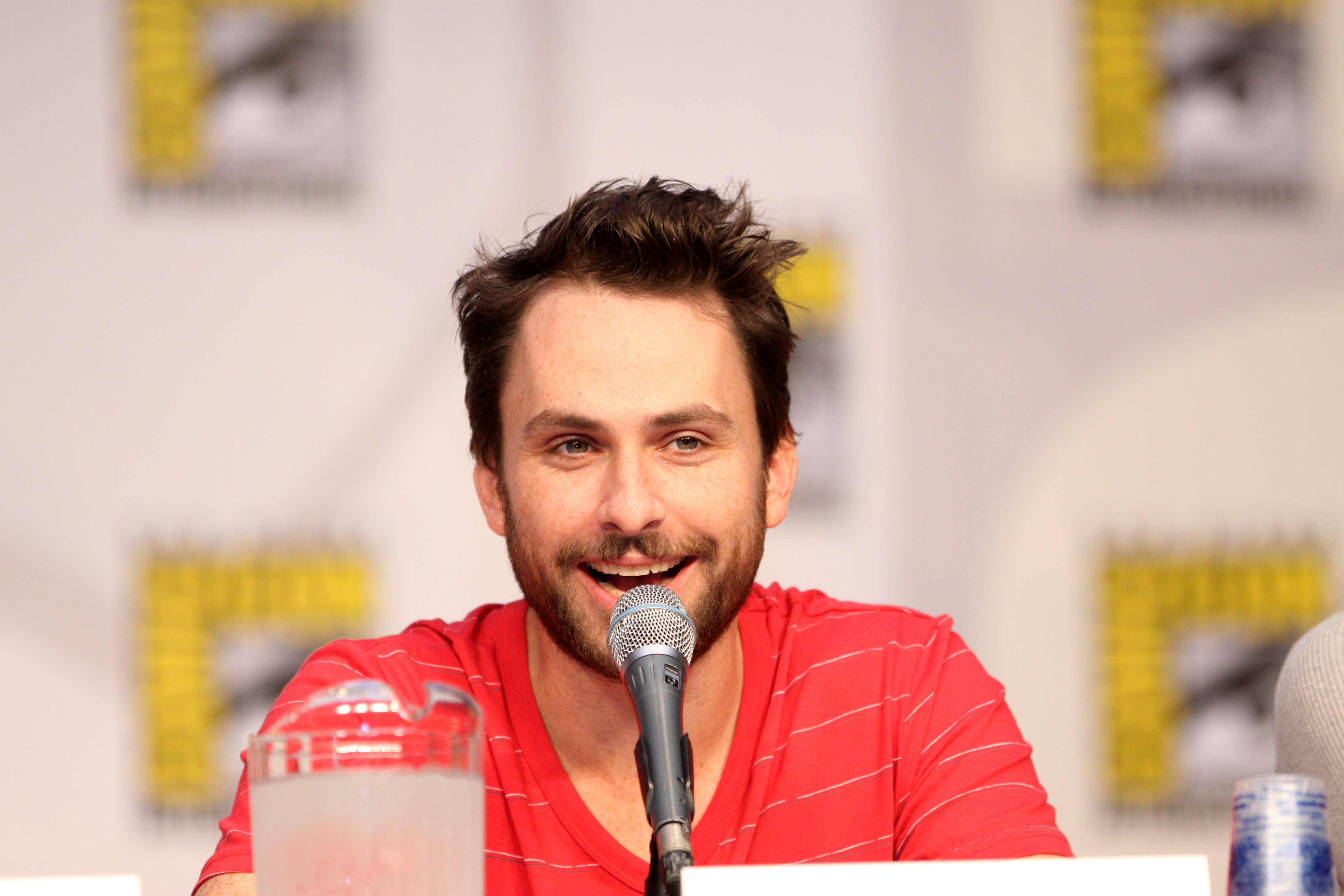This photo captures Charlie Day at a Comic-Con panel, seated behind a table with multiple blurry Comic-Con logos repeatedly printed on the banner behind him. Charlie Day is in a red t-shirt featuring thin white stripes and is holding a black and silver microphone positioned in front of him. To his left, a plastic pitcher of water is visible. He has brown hair, styled brushed back, and a short, brown beard that outlines his lips, jaw, and chin, connecting seamlessly with his hair. To his right, the corner of what appears to be a gray shirt or sweater of another person is visible, along with an upside-down plastic cup also positioned to his right. Charlie Day is captured smiling, embodying a relaxed and engaging presence at the event.